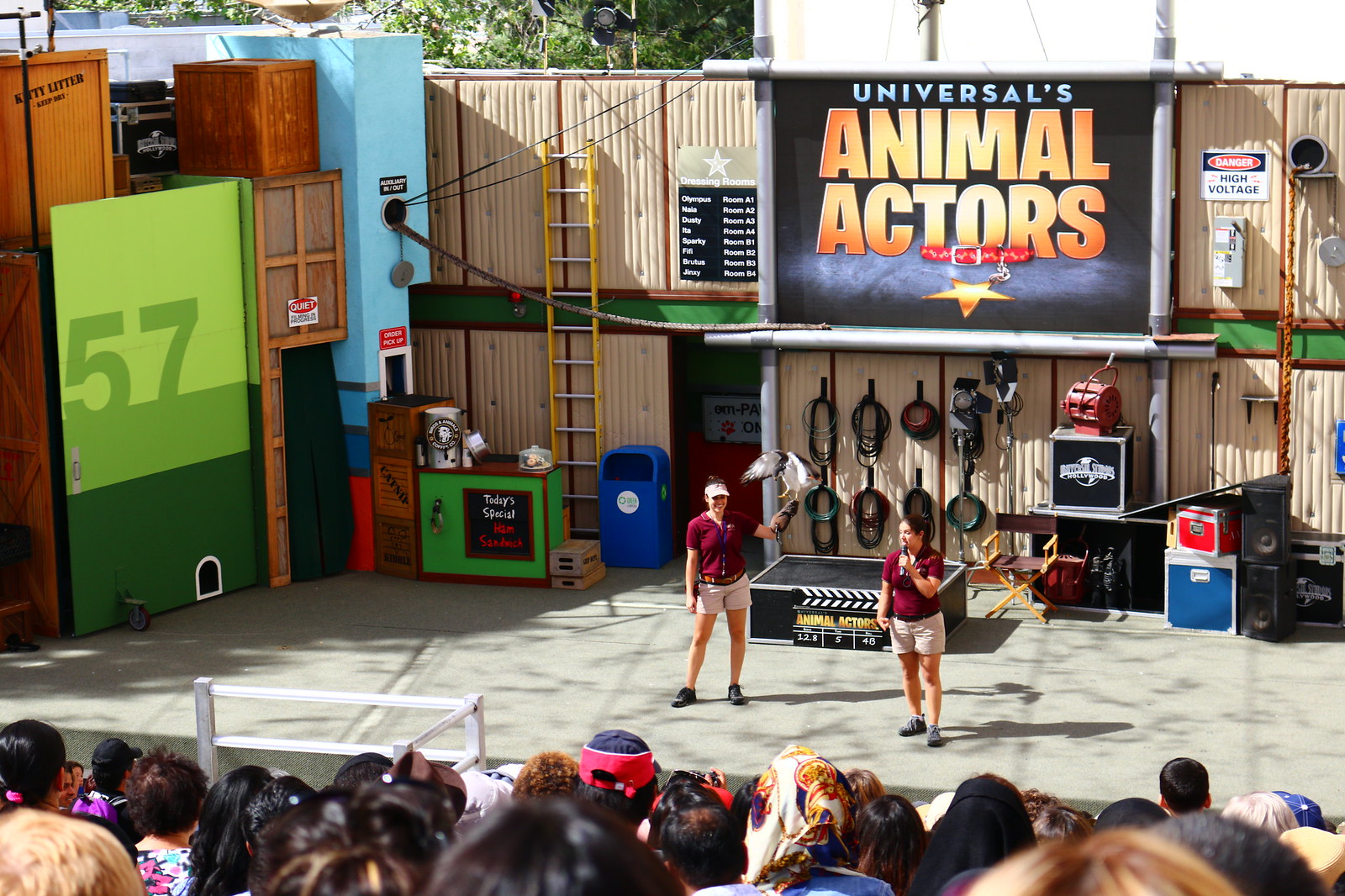In this detailed photograph taken at Universal Studios, we see a vibrant outdoor setting during the middle of the day. The central focus is a stage situated amidst a large crowd of spectators arranged in several rows at the bottom of the image. Two women, positioned centrally on the stage, are engaged in an animal show. Both women are dressed in maroon polo shirts and beige khaki shorts, complemented by dark shoes. One woman is smiling while holding a large bird, possibly a hawk, perched on her hand, while the other woman speaks into a microphone, likely sharing interesting facts about the bird.

Above the stage, there is a prominent sign reading "Universal's Animal Actors," adorned with a collar and a star emblem. The stage itself is equipped with various objects including ladders, drawers, a platform, and a director's chair. There's also a backdrop that features signs indicating dressing rooms, along with names of the animals, hinting at their roles in movies and shows. The vivid palette of colors in the image includes brown, black, pink, purple, blue, gray, white, tan, green, yellow, orange, red, and silver, enhancing the lively atmosphere of this amusement park attraction.